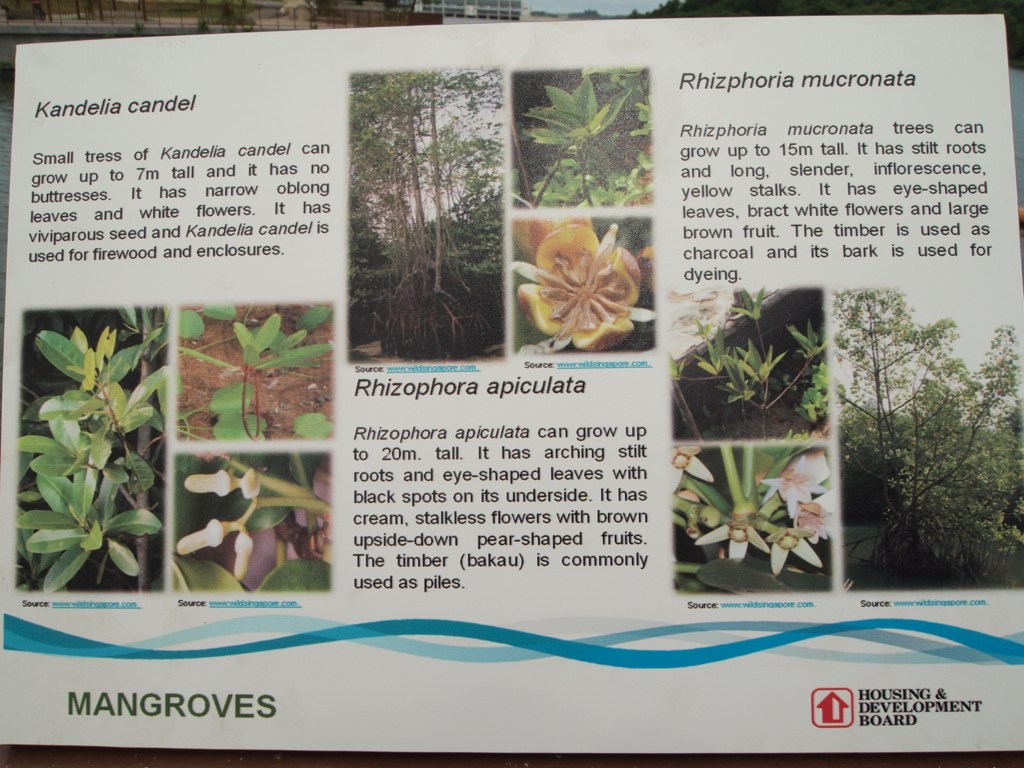This image displays a detailed informational sign, presumably located in a park or botanical garden, showcasing various plant species found in mangrove ecosystems. The title "Mangroves" is prominently printed in the bottom left corner, and a red house logo representing the Housing and Development Board is visible in the bottom right corner. 

The sign provides comprehensive descriptions of three plant species. The first is Candelia candel, described as a small tree that can grow up to seven meters tall, characterized by its narrow oblong leaves and white flowers. It has viviparous seeds and is utilized for firewood and enclosures. 

Adjacent to this are sections dedicated to Rhizophora apiculata and Rhizophora mucronata, each accompanied by images depicting the plants' leaves and buds. The visually rich display aims to educate visitors about these integral components of the mangrove ecosystem.